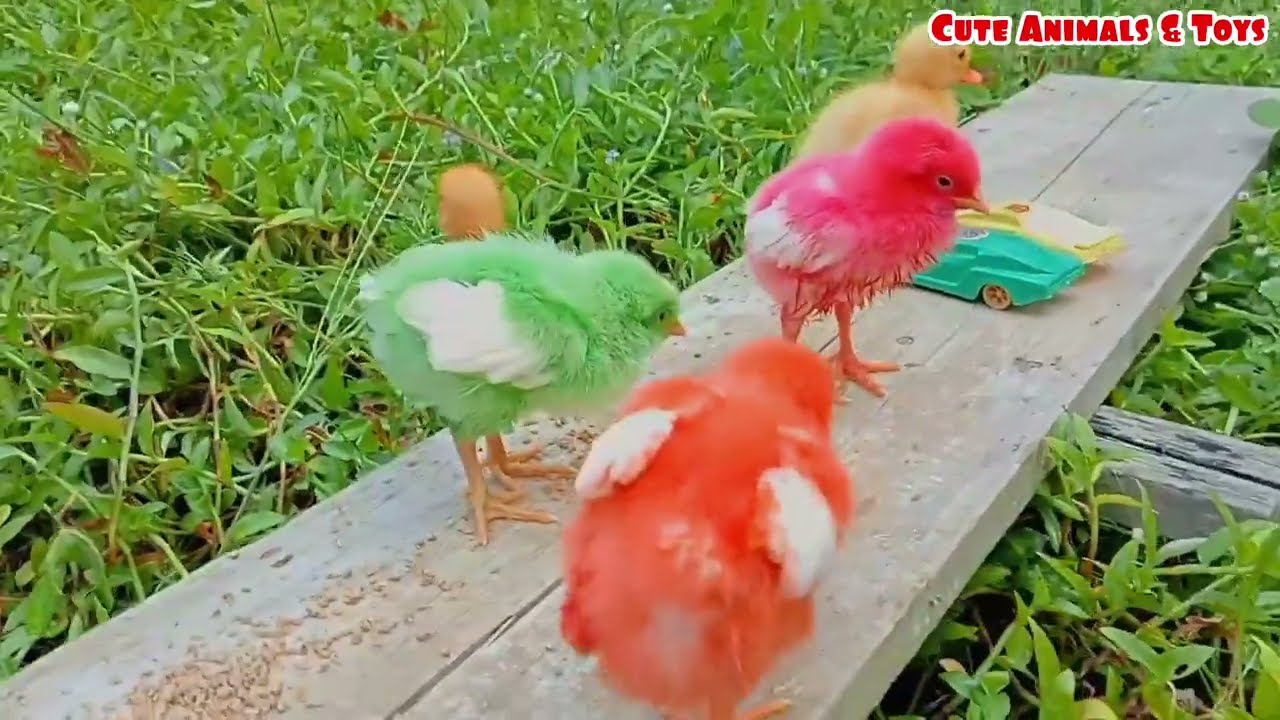The landscape-oriented color photograph showcases a whimsical scene of baby birds standing on a weathered bench amidst green vegetation. Four baby chicks, dyed in vibrant shades of light green, pink, and orange, each with white wings, share the bench with a naturally-colored yellow duckling sporting a distinct duck beak. Scattered grains keep them engaged on the worn wooden surface. At their feet are two toy cars, one green and yellow and the other aqua, adding a playful touch to the setup. The bench is surrounded by verdant ground cover, emphasizing the natural yet charmingly artificial setting. Overseeing this adorable tableau, red lettering in the top right corner proclaims "cute animals and toys," suggesting a playful interpretation of the scene's reality.